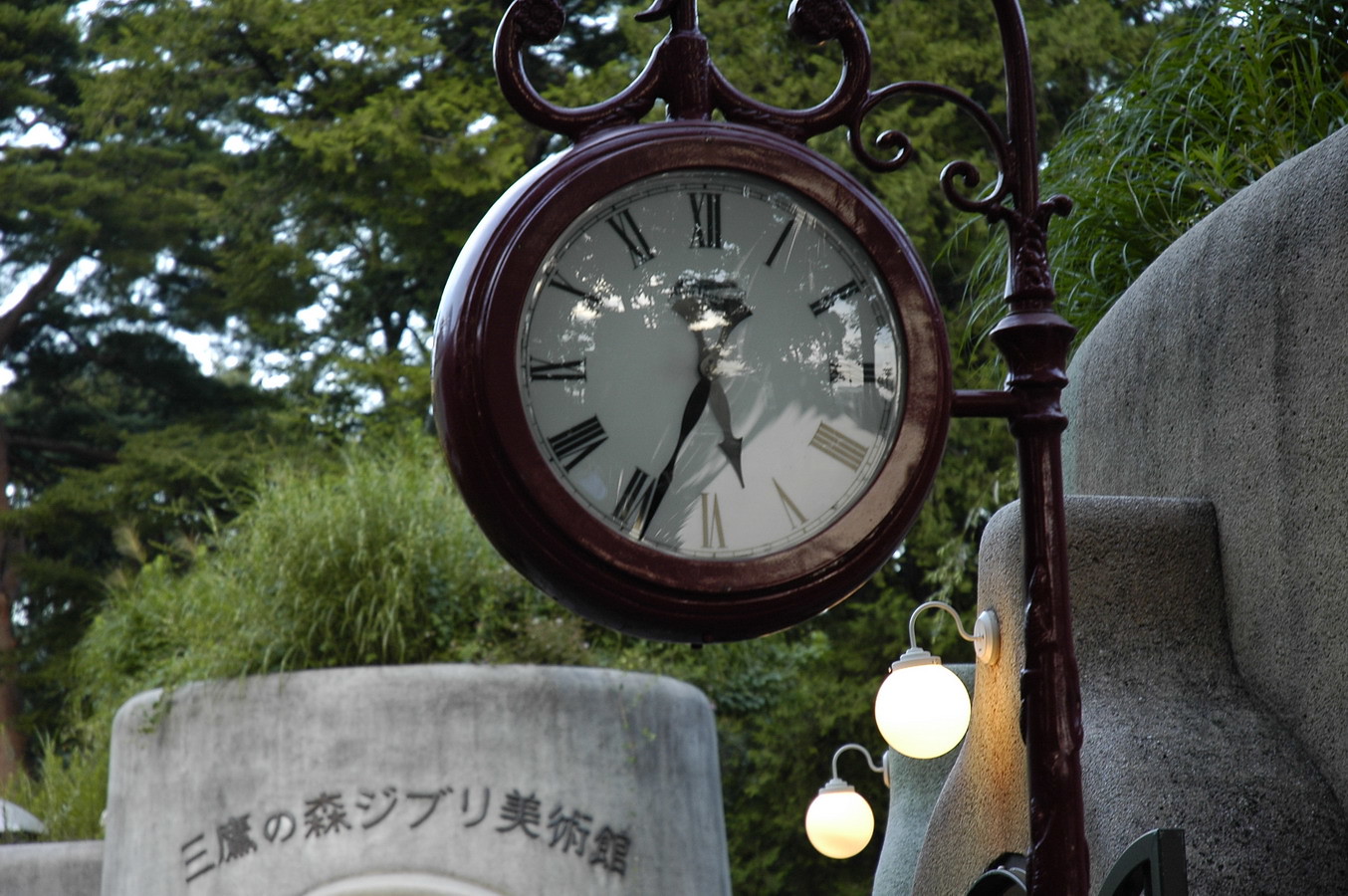This image showcases an ornate, vintage clock mounted on a wrought iron stake. The stake is a brown-colored pole adorned with decorative scallops that ascend towards the top where the clock is suspended. The clock, featuring a white face with elegant Roman numerals, hangs securely from the upper portion of the scalloped design, with additional support provided by a small side bar. 

The outdoor setting bathes the scene in natural light, with reflections of sunlight and surrounding trees visible on the clock's face. In the foreground, a gray gate or barrier partially obscures the view, adding a sense of depth. 

In the background, modern lights, which are affixed to a concrete wall or structure, illuminate the scene. The structure also bears Asian script, which intriguingly resembles the upper portion of a tombstone. Completing the picturesque environment are lush trees and bushes, framing the entire composition beautifully.